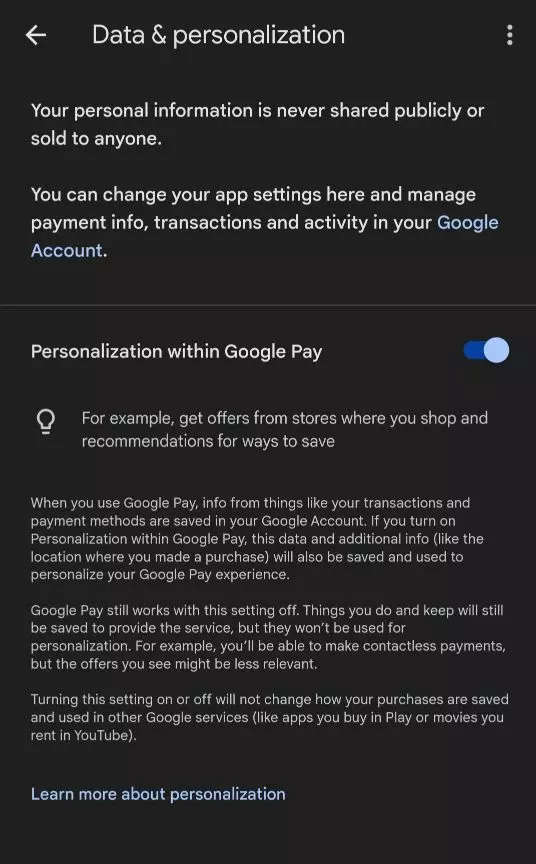The image displays a section of Google Settings under the "Your Data & Personalization" tab. At the top of the screen, the title "Your Data & Personalization" is prominently displayed, with a left-pointing arrow on the left side for navigating back, and a vertical ellipsis (three dots) on the right side for accessing page options.

The main body of the screen contains a reassuring message: "Your personal information is never shared publicly or sold to anyone." Below this, users are informed they can manage their app settings, payment information, transactions, and account activity.

Further down, the screen shows the "Personalization with Google Pay" option, which is currently enabled, indicated by a blue toggle switch. This section includes a light bulb icon and a tooltip explaining the benefits: "For example, get offers from stores where you shop and recommendations for ways to save." Additionally, it clarifies that when you use Google Pay, transaction and payment method information is stored in your Google account. 

If personalization is turned on, additional details like purchase locations will also be saved to tailor the Google Pay experience. Turning this feature off will still save your transactions to provide services, but they won't be used for personalized offers or recommendations. It is noted that this setting does not affect how purchases are used in other Google services, such as apps bought on the Play Store or movies rented on YouTube.

At the bottom of the screen, there is a link labeled "Learn more about personalization" for users who want more detailed information on how their data is used.